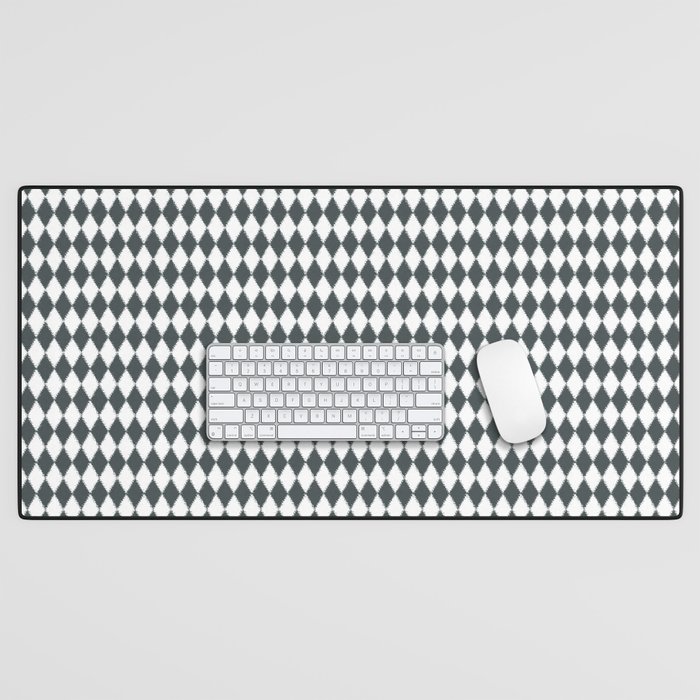An overhead photograph captures a modern and minimalist white wireless keyboard and a sleek, buttonless white wireless mouse, presumably from Apple, set against a sharp and visually striking black and white diamond-patterned mat. The mat, which covers the entire rectangular frame, features rows of alternating white and charcoal gray diamonds, creating an almost grayscale illusion due to the contrasting colors. The diamonds are bordered by a distinctive dark black edge. The keyboard is placed approximately two-thirds of the way down the mat and is centered, while the mouse rests to the right of the keyboard at an angle, positioned from the top left to bottom right. The overall composition is clean and devoid of color, emphasizing the interplay between the stark black and white elements.